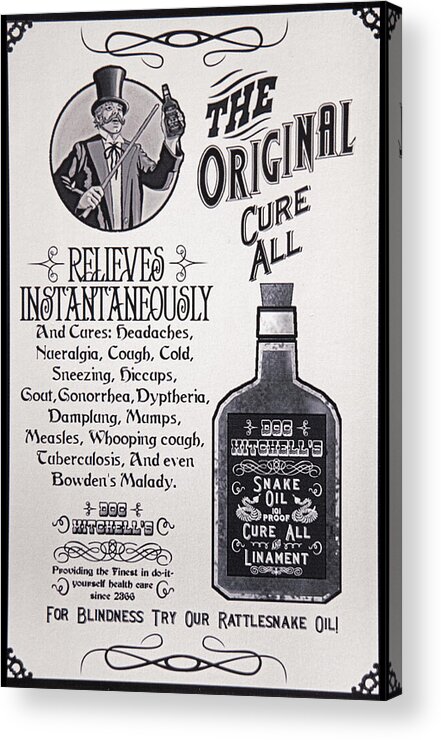This is an old-fashioned, black-and-white framed advertisement for "Doc Mitchell’s Snake Oil 101 Proof Cure-All Liniment." The portrait-oriented canvas, designed to look aged with ornate embellishments in the corners and a thin black border, is printed on a slightly off-white or gray background. In the upper left corner, a circular illustration depicts a man in a top hat and suit, sporting a monocle and holding both a cane and a bottle of the cure-all. Beside him, bold text reads "The Original Cure-All." Below, a large image of the product bottle with a cork is prominently displayed. The advertisement boasts in a vintage font that the product "Relieves instantaneously and cures headaches, neuralgia, cough, cold, sneezing, hiccups, gout, gonorrhea, diphtheria, damp lung, mumps, measles, whooping cough, tuberculosis, and even Bowden's malady." Additional text humorously suggests that for blindness, one should "Try our Rattlesnake Oil." The ad exudes a nostalgic charm, harking back to the early 1900s with its stylized design and detailed presentation.